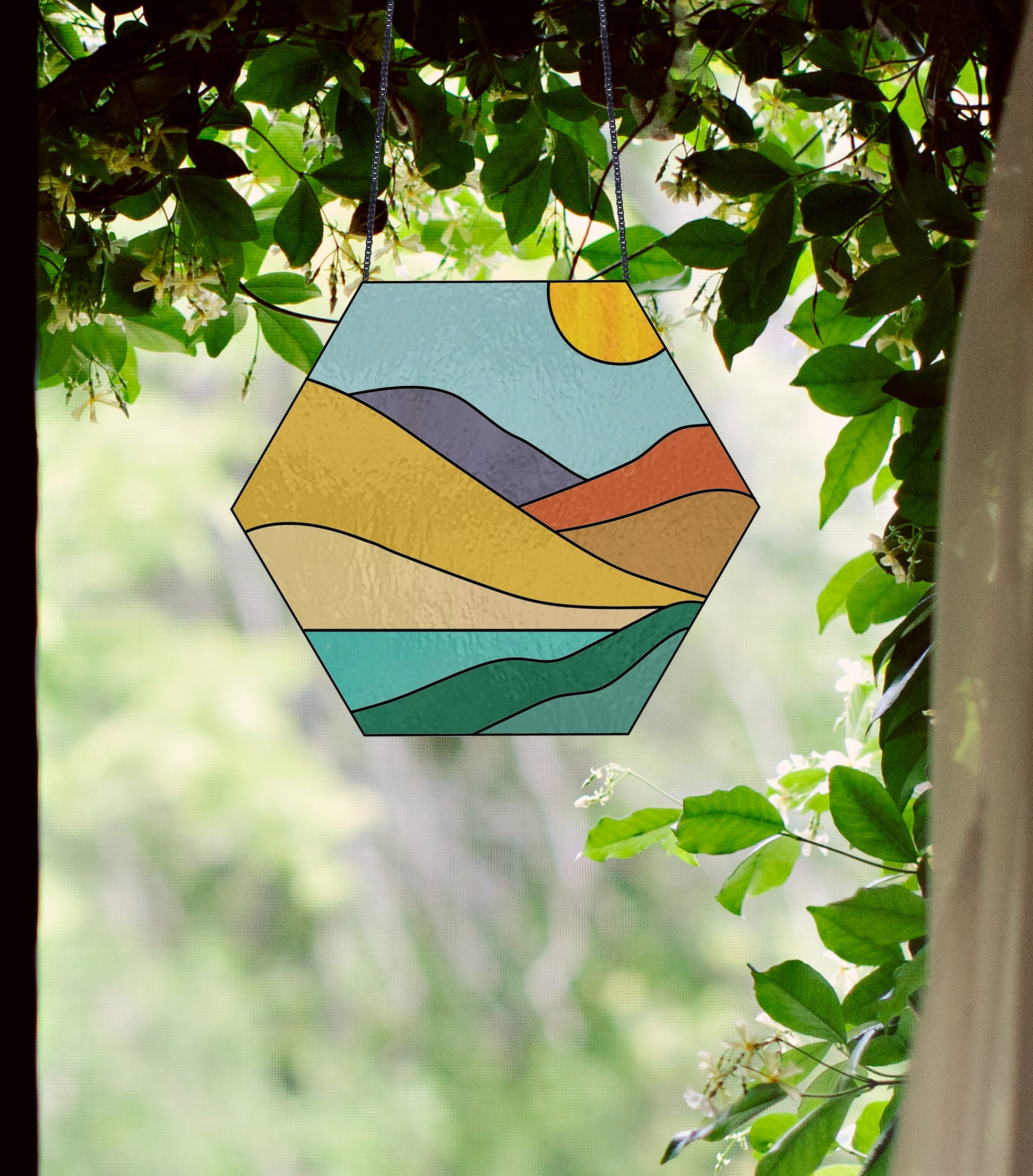The image features a hexagon-shaped stained glass ornament depicting an abstract outdoor scene. Suspended by two intricate black chain links, the glass piece hangs in front of a house. The artwork showcases a series of colorful, curved layers resembling mountain ranges. These layers include shades of green, yellow, beige, orange, brown, teal, and dark teal. In the upper right corner of the glass, a yellow circle symbolizes the sun set against a sky blue background. Surrounding the ornament are lush green leaves and vines, accompanied by white flowers in the foreground. The background is a blurry mix of green, hinting at more trees and foliage. On the right side, there is a brown strip that appears to be a curtain and a black streak on the left. The vibrant colors and detailed patterns create a minimal yet striking visual set in a natural outdoor environment.